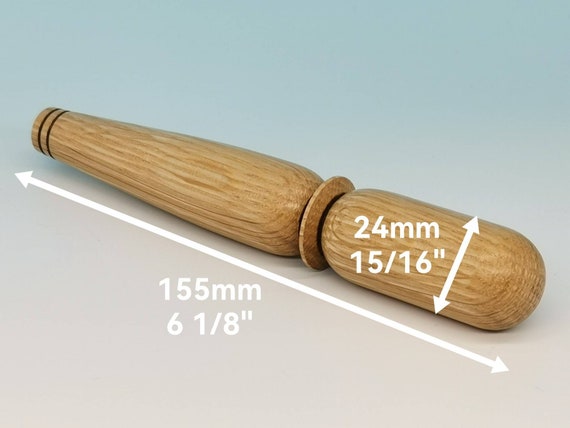The image, presented in landscape mode, features a wooden tool displayed against a gradient background that transitions from aqua at the top to cream at the bottom. The focal point of the image is a wooden object that is slimmer on the left and gradually widens towards the right, appearing slightly pointed and angled upwards to the left. This tool is marked with two brown circular notches near its left end and a connecting wooden ring towards the middle, which links two distinguishable sections. The left section appears cylindrical with notches, while the right section, which is more oblong, resembles a handle. The entire wooden object, characterized by its light brown layered texture, is annotated with white arrows indicating its dimensions: a length of 155 millimeters (6 1/8 inches) and a maximum width of 24 millimeters (15/16 inches).